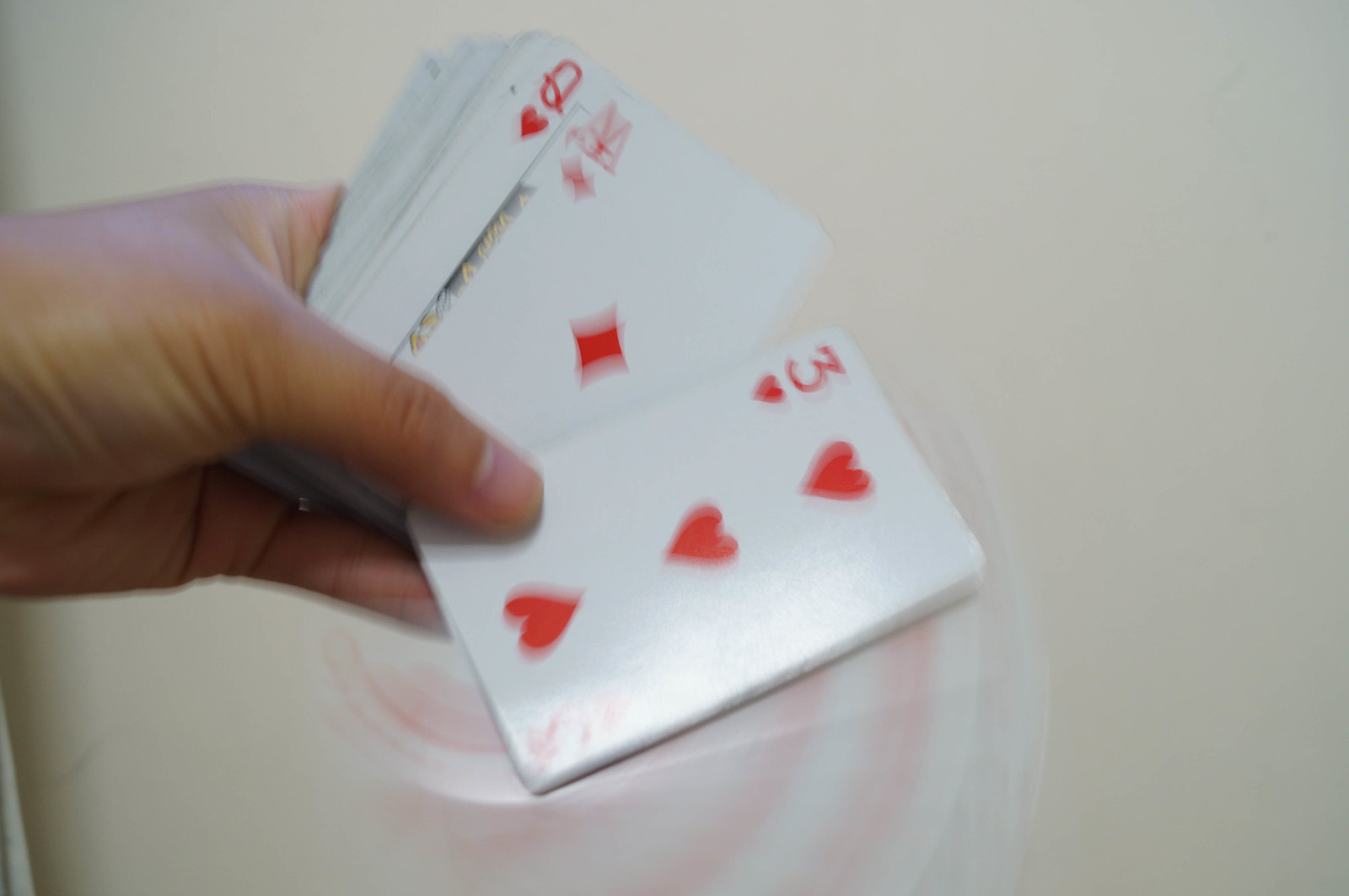This real-life photograph features a light brown, right hand extending from the left side of the frame, holding a thick stack of playing cards. The image cuts off just before the wrist, focusing solely on the hand and the cards. The cards are prominently displayed for the viewer to see: the three of hearts, which is red, is being slid almost completely off the deck, revealing the ace of diamonds beneath it. The ace of diamonds is also slightly displaced, allowing a glimpse of the queen of hearts underneath. Beyond these three, the remaining cards, presumably forming a full deck, are not visible.

The background is a soft, blurry eggshell white, with no distinct features or elements in focus. Notably, there is a blur or motion effect around the three of hearts, suggesting the card was swiftly moved or rotated. This effect manifests as faint red and white streaks near the card's surface, aligning with the positioning of the hearts and numerical three.

Overall, the photo captures the dynamism of card movement and the intricacies of the hand holding them, set against a simple, unobtrusive background.